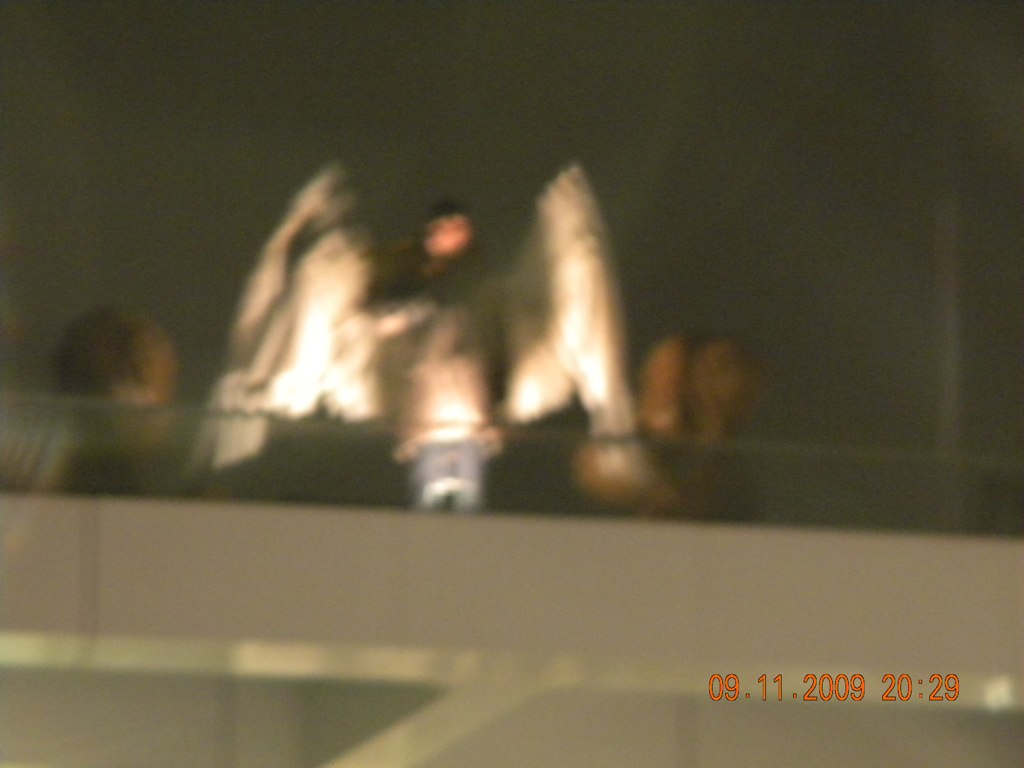The image is a blurry, low-resolution nighttime photograph, likely taken with an unstable camera. The top two-thirds of the photo are dark, suggesting a view of the night sky. The bottom section contains a glass-lined structure that resembles the edge of a balcony or a mantle with white beams for support. At the center of the image, slightly to the left, sits an angel-like figure with dark gray and white wings, illuminated from below. The figure appears to have a brown body with a black splotch and a peach splotch above it. Surrounding the figure, there might be additional blurred shapes that could be statues or people, and a distinct, small red light blob can be seen above the central figure. On the right-hand side, a timestamp in red text reads "09.11.2009 20:29," anchoring the photograph in time. The scene evokes an ethereal atmosphere against the stark contrast of the black sky above.